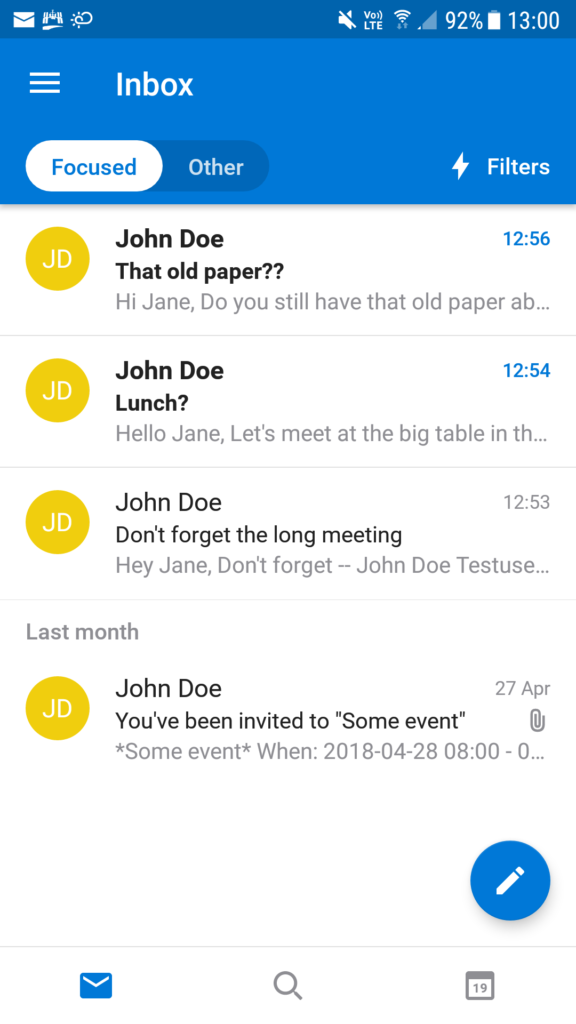The image depicts a messaging inbox, segmented into two tabs labeled "Focused" and "Other." The top part of the interface is blue, with the section headers in white. When an item is highlighted, the background turns blue and the letters switch to white, while unhighlighted text appears in black.

Prominently displayed is a message from "John Doe," shown against a yellow background with white text reading "John Doe." Several snippets of messages are visible:

1. A message from "John Doe" to "Jane" reads: "Hi Jane, do you still have that old paper?" This message is cut off before the end.
2. An earlier message from John Doe says: "Lunch? Hello Jane, let's meet at the big table..." This message is also cut off and incomplete.
3. Another message: "Don't forget the long meeting. Hey Jane, don't forget the test..." with a timestamp reading 12:53 PM from last month.
4. The final visible message is an invitation to an event from "John Doe."

The overall design suggests an organized messaging system, where more recent messages appear at the top, and older messages stack below. The layout employs a clear structure with highlighted interactions altering the color schema to facilitate user navigation.